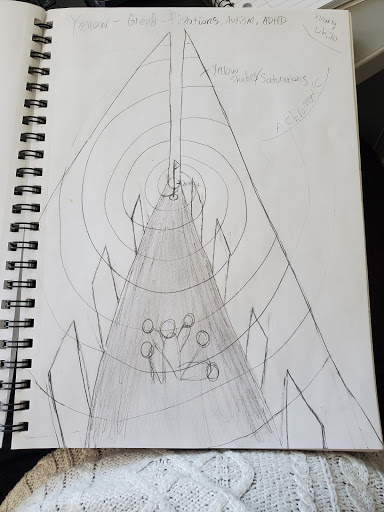A detailed pencil drawing on an open spiral notebook, resting atop a lace sweater on a person's lap, occupies most of the image. The edge of a table is partially visible at the top of the photo. The drawing portrays a long, simplistic hallway with three evenly spaced doorways on each side. A rudimentary humanoid figure stands at the center of the hallway, featuring a round head, circular hands, and tubular arms and body. Handwritten words appear at the top of the page, including "yellow," "greed," "fixations," "autism," and "ADHD," along with some other illegible text.